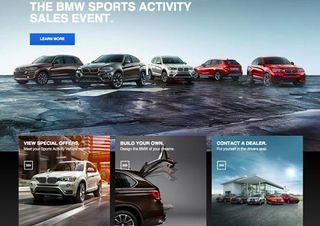The image prominently features a BMW promotional event for their Sports Activity Sales. In the upper left corner, bold white capital letters announce "BMW Sports Activity Sales Event." Directly beneath this text, a solid dark blue rectangle displays the phrase "LEARN MORE" in white capital letters. Below this, five BMW vehicles are showcased from left to right in the following colors: dark brown, dark gray, light gray, red, and another red, all positioned against a wet tar surface. The backdrop shows a gradient sky transitioning from white at the horizon to a medium pale blue at the top.

At the bottom of the image, there are three clickable thumbnails. The left thumbnail depicts a silver SUV driving on wet pavement, its shadow visible on the ground. It features the text "VIEW SPECIAL OFFERS" in white capital letters, accompanied by a square with a white border—though the content inside the square isn't clear.

The middle thumbnail displays a vehicle with its trunk open, revealing only a third of the car. The top left corner reads "BUILD YOUR OWN" in white capital letters, with additional smaller text below that is not legible.

The right thumbnail says "CONTACT A DEALER" in white capital letters and shows an image of a blue sky with wispy clouds. This thumbnail also includes a scene with a house or canopy area, showcasing several cars: a silver one, a black one, and two red ones.